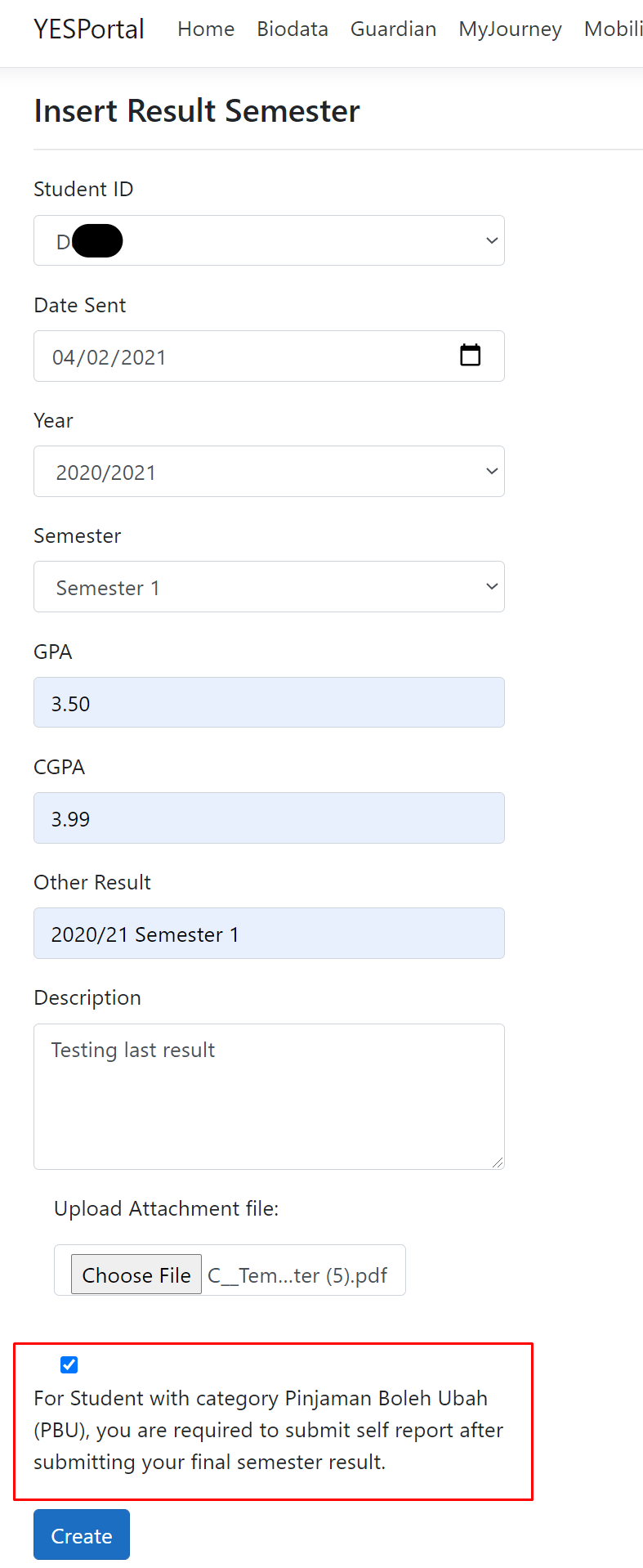**Detailed Image Description: YES Portal Student Result Submission Interface**

The image on the smartphone screen displays a student portal interface, specifically the result submission section of the YES Portal. The background of the interface is predominantly white, creating a clean and professional look. 

**Top Navigation Bar:**
At the top of the screen, there is a black navigation bar with six tabs or clickable categories. From left to right, the categories are labeled:
1. YES PORTAL (in all caps)
2. HOME
3. BIODATA
4. GUARDIAN
5. MYJOURNEY
6. MOBILI (likely an abbreviated or cut-off form of "mobility")

**Main Content Area:**
Underneath the black navigation bar, there is a light gray bar, providing a sub-header or demarcation. Below this, in bold black letters, is the heading "INSERT RESULT SEMESTER."

**Input Fields and Drop-Down Menus:**
Following the heading, there are a series of interactive fields, primarily in the form of drop-down menus and input bars with light blue backgrounds:
1. **STUDENT ID:** The drop-down menu shows a selected student ID beginning with "D," with the rest of the ID redacted.
2. **DATE SENT:** This field includes a calendar icon, displaying the selected date April 2, 2021, presented as "04-02-2021."
3. **YEAR:** The selected academic year in the drop-down menu is "2020-2021."
4. **SEMESTER:** The selected semester is "Semester 1."
5. **GPA:** The GPA field displays a value of "3.5."
6. **C GPA:** Shows a cumulative GPA of "3.99."
7. **OTHER RESULT:** This field indicates "2020-21 Semester 1."

**Description and File Upload:**
Below these fields, there is a "DESCRIPTION" box containing the text "TESTING LAST RESULT." This box provides ample space for additional text, with the ability to drag the bottom right corner to resize it.

Further down, there is an "UPLOAD ATTACHMENT FILE" section. Within this section, a gray rectangle labeled "CHOOSE FILE" displays the selected file "c..term..ter (s.pdf)," indicating a PDF file for the semester.

**Submission Note and Action Button:**
At the bottom of the screen is a red-outlined section with a notification for students categorized under "PINJAMAN BOLA UBA (P.B.U.)." It states that these students are required to submit a self-report after submitting their final semester results. There is also a small blue box with a white check mark, suggesting a completed action or a required task.

The final element present is a blue clickable button labeled "CREATE," indicating the option to submit or finalize the entered data.

This detailed description outlines the student portal's various elements, providing a comprehensive overview of the interface and its functionalities.